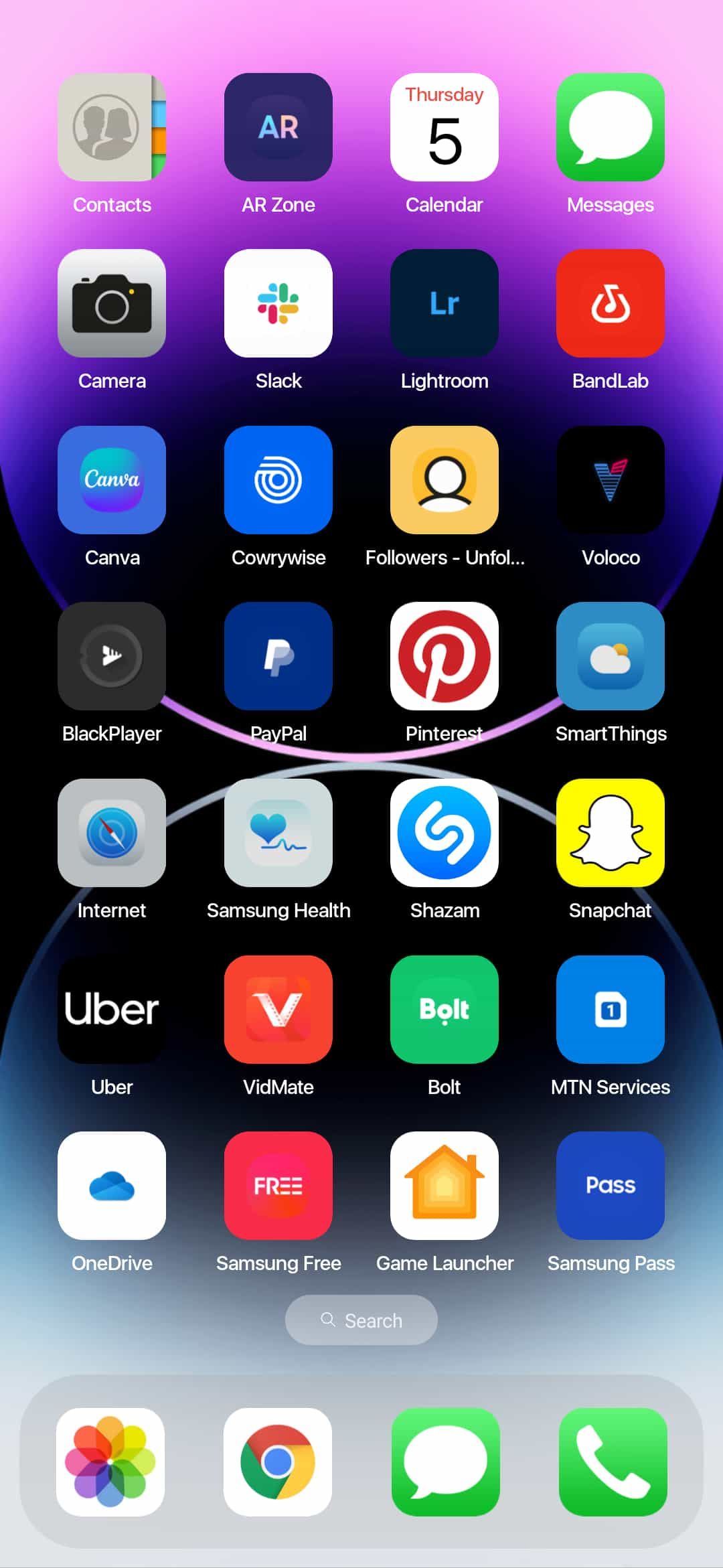This is a detailed screenshot of a smartphone's home screen. The wallpaper is a gradient that starts with a pale pink at the top, transitioning into purple, then blue, and finally black. From the bottom, the gradient begins as pale gray, shifts to blue, and merges into black in the middle, creating a striking background effect. 

The home screen is organized into seven rows, each comprising four app icons, making a total of 28 apps displayed. The apps are arranged as follows:
1. Contacts, ARZone, Calendar, Messages
2. Camera, Slack, Lightroom, BandLab
3. Canva, Cowerywise, Followers-Unfollow, Voloco
4. Blackplayer, PayPal, Pinterest, SmartThings
5. Internet, Samsung Health, Shazam, Snapchat
6. Uber, Vidmate, Bolt, MTN Services
7. OneDrive, Samsung Free, Game Launcher, Samsung Pass

At the bottom of the screen, there are four primary shortcuts: Instagram, Google Chrome, text messages, and phone calls.

Overall, the meticulously organized layout and gradient wallpaper create a visually appealing and highly functional home screen.